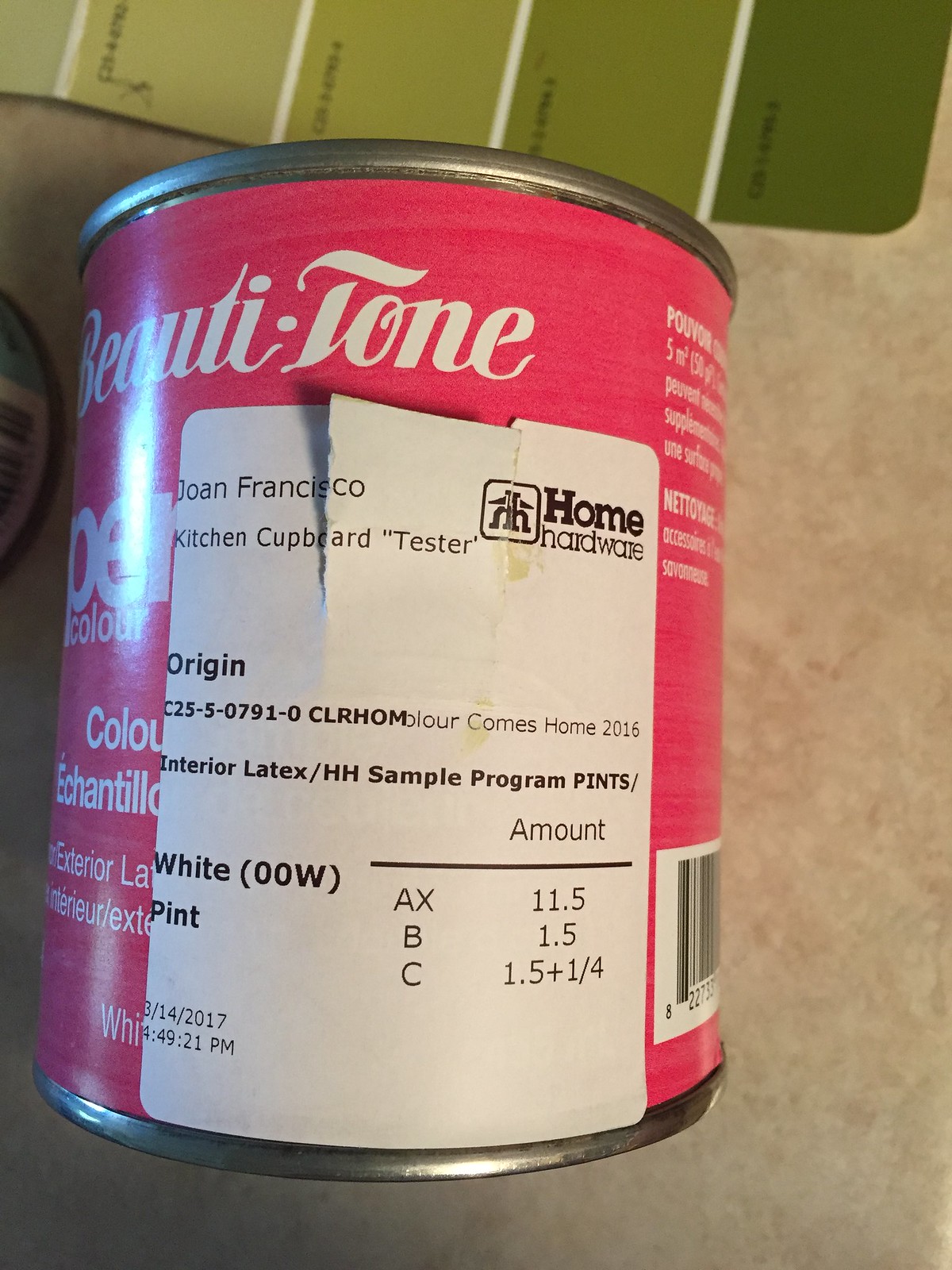The image portrays a scene centered around a small, reddish-pink paint can resting on its side, prominently displaying a 'Beauty Tone' label. Key details on the label include its origin from Home Hardware and the words, "Joan Francesco Kitchen Cupboard Tester." The label also notes it is an interior latex paint and includes specifications such as 'White Pint'. The date and time, 03-14-2017, 4:49:21 PM, are printed at the bottom of the label. Surrounding the main paint can is a selection of olive green paint samples that transition from light to dark, positioned at the top of the image. They collectively rest on a speckled surface that is whitish-tan in color, likely that of a table. On the far left, another paint can is partially visible, with its label contributing to the backdrop but not drawing the immediate focus away from the centrally highlighted can.